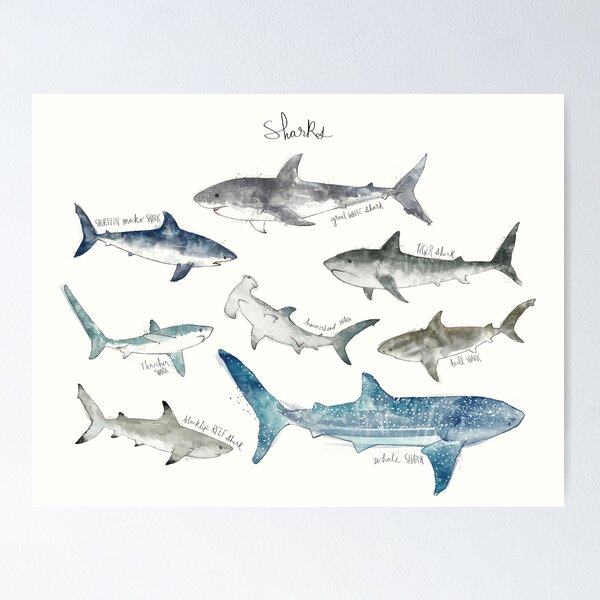This image showcases a detailed, hand-drawn illustration of various types of sharks on a white piece of paper, adorned with watercolors and outlined in black. The title at the top reads "Sharks" in bold, aggressive writing. Below the title, there are meticulously labeled depictions of different shark species, arranged in proportion to their actual sizes. Prominently, the great white shark is featured and clearly marked. To its left is another shark, presumably the thresher shark, though its label is less visible. To the right, the tiger shark is depicted, and below it, the hammerhead shark is positioned. Adjacent to the hammerhead shark on the right is the bull shark. Below the bull shark resides the whale shark, the largest of all, distinctly blue with white dots. To its left lies the blacktip reef shark, completing this rich marine tableau.